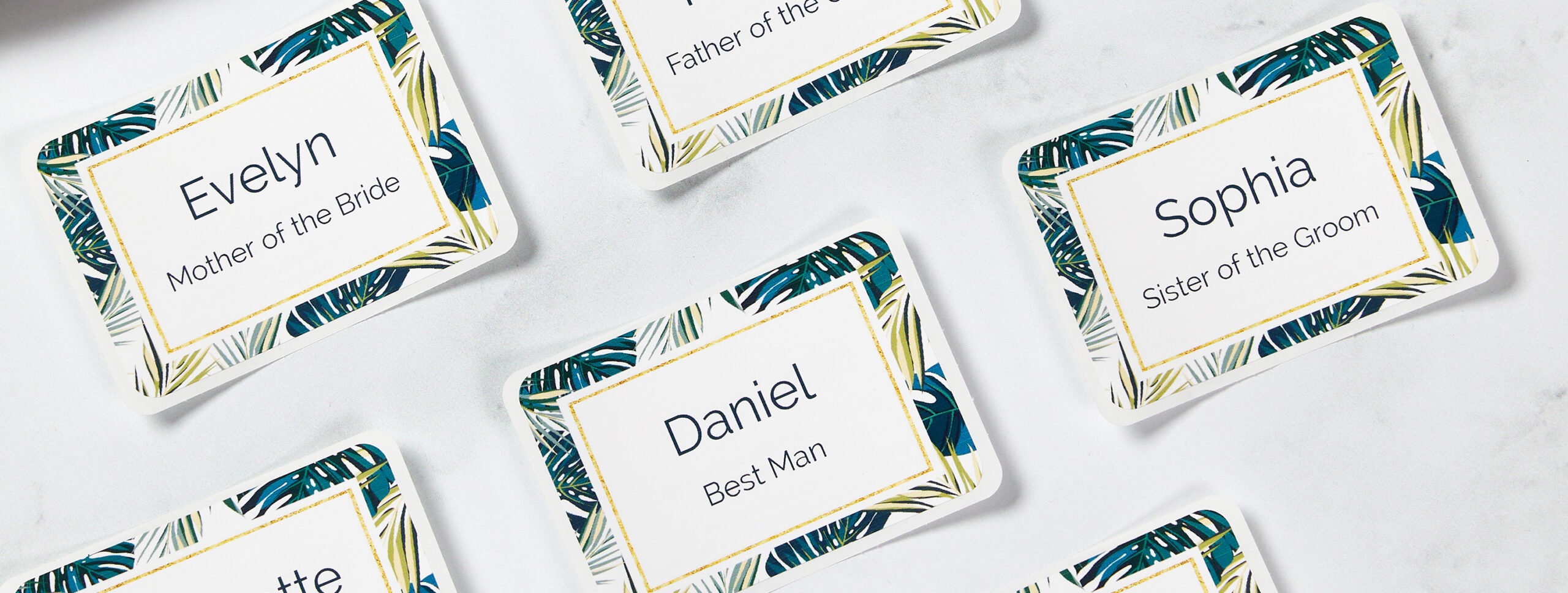The image displays an array of wedding name tags meticulously arranged on a white background, each set at a diagonal angle ascending towards the right. Each name tag features bold black text with the names more prominent than titles. Notably, the name tags have a decorative border featuring an assortment of tropical leaves and a yellow inner border, adding a vibrant touch. Featured name tags include "Evelyn, Mother of the Bride" positioned at the top left, "Daniel, Best Man" towards the bottom middle, and "Sophia, Sister of the Groom" to the right of Daniel’s tag. Partially obscured tags for the "Father of the Bride" are visible at the top middle, bottom left, and near the bottom right, indicating additional roles crucial to the wedding. These name tags are designed to help attendees identify significant family members and their roles in the wedding celebration.